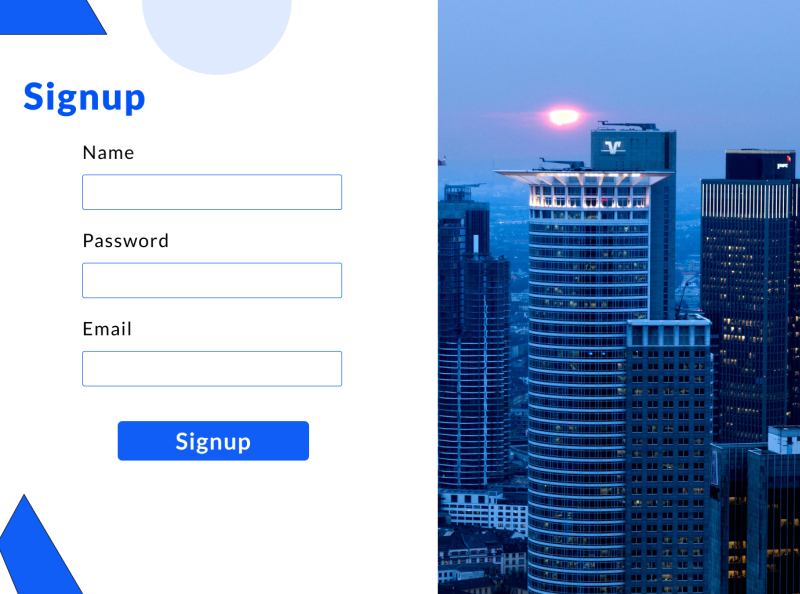This image depicts a stylish sign-up page layout. On the right side, there's a scenic photograph of a city skyline at dusk. Dominating the scene are several skyscrapers against a gray sky, with the focal point being an orange sun setting just to the left of the tallest building in the center. The setting sun casts a gentle glow, creating a serene urban landscape.

On the left side of the image is the sign-up form set against a white background. In the top left corner, there's a blue bar with a partial blue circle adjacent to it. Below this, the word "Sign-Up" is written in blue text. The form includes three input fields: one labeled "Name" for entering the user's name, another labeled "Password" for entering the user's password, and a third labeled "Email" for entering the user's email address. Beneath these fields is a prominent blue "Sign-Up" button with white text. Additionally, in the bottom left corner, there is a small blue bar shaped like a trapezoid. The overall design is clean and modern, effectively guiding the user through the sign-up process with a blend of visual appeal and functionality.